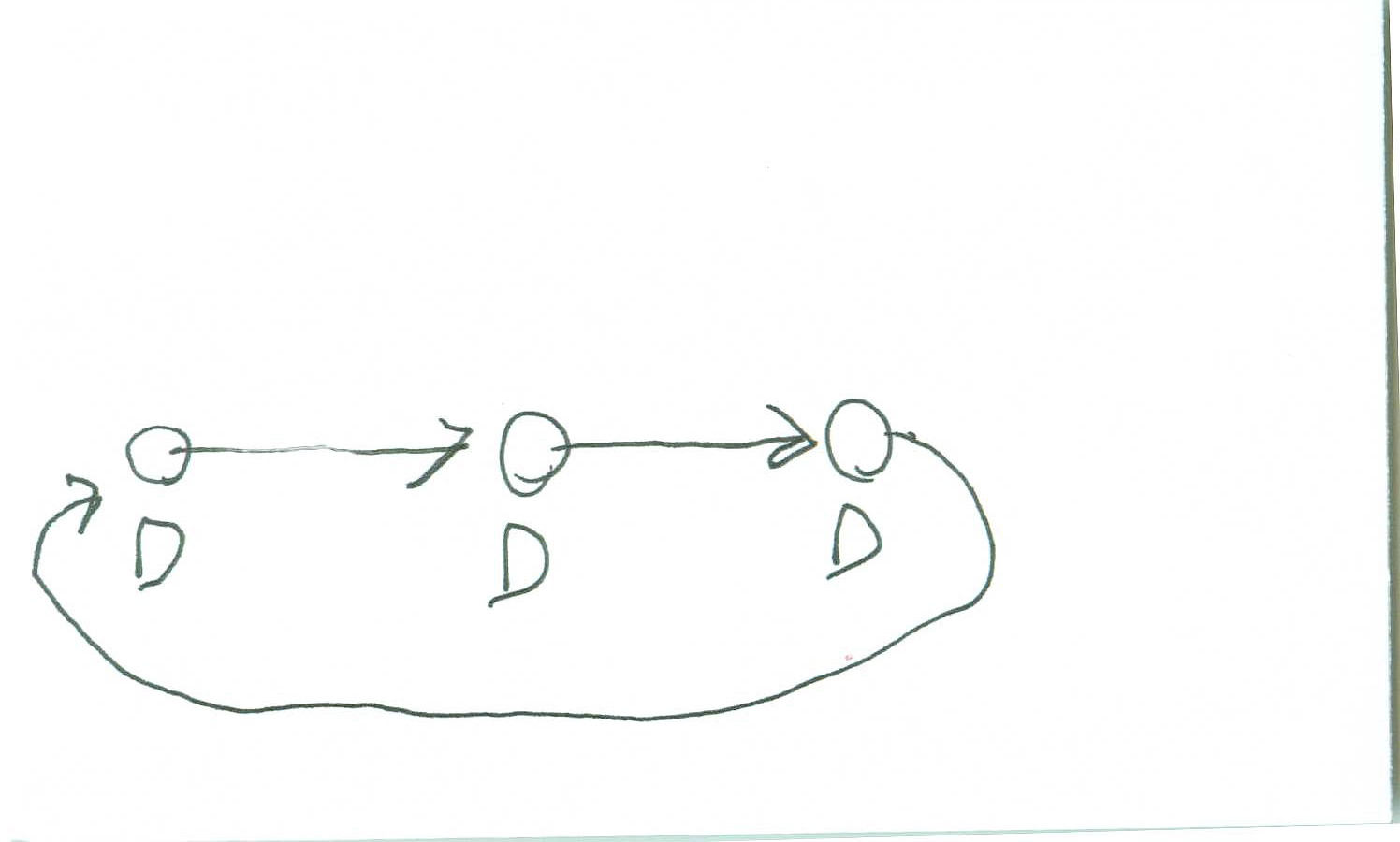A simple hand-drawn diagram is sketched on a piece of paper using pen or pencil in a greenish-black hue. The drawing features three roughly drawn circles, each spaced approximately an inch and a half apart. Lines with arrowheads indicate direction, connecting the circles from left to right: one line extends from the leftmost circle to the middle circle, and another from the middle circle to the rightmost circle. An extended, swooping line arcs to the right and then downward from the third circle, looping around several times before ending with an arrow pointing back to the first circle. Underneath each of the three circles, the capital letter "D" is crudely drawn. The overall diagram depicts a continuous flow from one circle to the next, ultimately looping back to the beginning.